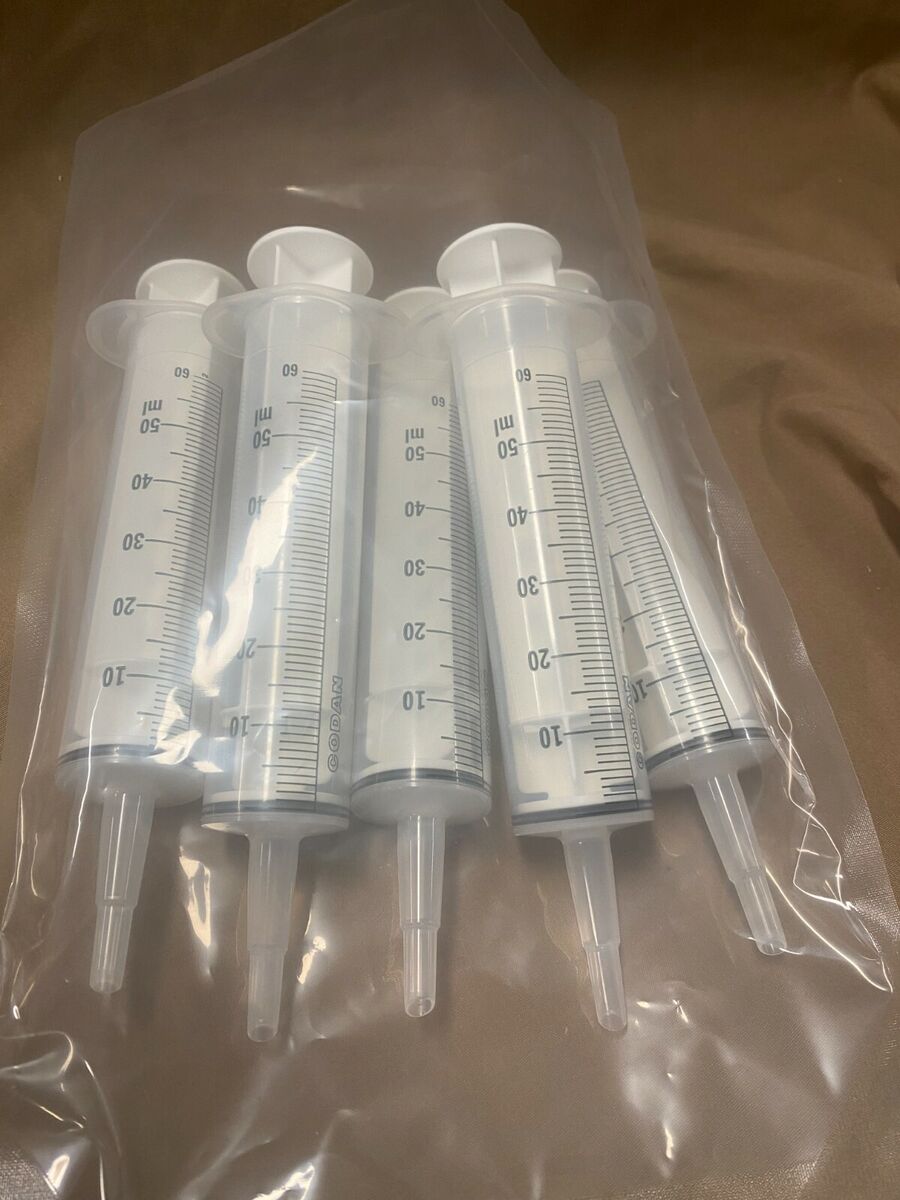In this detailed photograph, we observe five identical, unused syringes housed within a clear, unsealed plastic bag, resting on a piece of brown cloth adorned with visible folds. Each syringe is made of clear plastic with white plungers and is devoid of needles, indicating a possible alternative use such as for feeding. These syringes are graduated with black measurement markings, featuring numbers every 10 milliliters—from 10 up to 60, although the numbers 10 through 50 are more prominently displayed. The syringes lie tip-down within the bag, which reflects overhead lighting, casting shadows and glimmers on the cloth beneath. This careful arrangement and the visibility of precise details within the bag highlight the clean and orderly state of the equipment, suggesting its readiness for use.